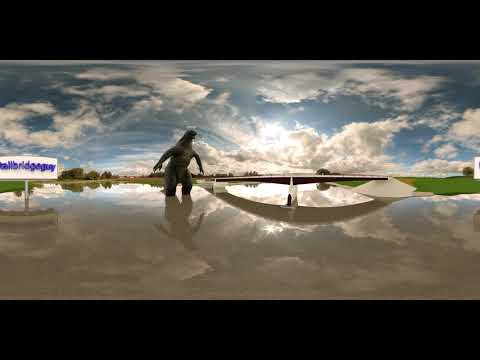In this outdoor scene depicted in the image, we observe a monster-like, Godzilla-esque creature with a human-like structure, standing ankle-deep in muddy water. This creature, featuring two arms and legs, is positioned slightly off-center to the left. The backdrop includes a white bridge spanning a body of water or a bay, with a green patch of grass visible on the right side. To the creature’s right, there's a white sign with blue letters that says "Tallbridge guy," attached to a silver pole. Surrounding this central figure, grass and various statues or signs are submerged in the water, indicating a flooded area. The distant background is marked by a tree line stretching across the image. Above this scene, the sky is largely overcast with gray and white clouds, though hints of blue sky and sunlight peek through. The entire image is framed by a black border, providing a cinematic feel.